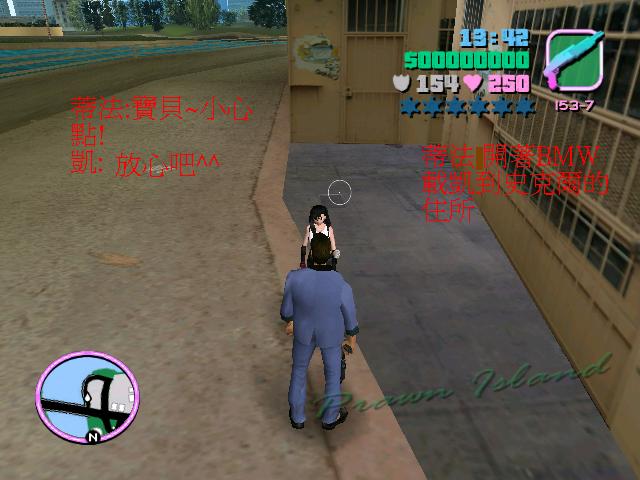The screenshot captures a moment from a Chinese video game, potentially resembling a scene from "Grand Theft Auto: Vice City." The central character, facing away from the player, wears a medium blue suit and holds a shotgun in his right hand. Positioned in front of him is a woman with black hair wearing a white dress. They appear to be standing on a pavement beside a tan building, possibly near a highway or parking garage. The screen features Chinese text in several locations: three lines to the upper left and additional text in the middle right. In the upper right corner is a stylized HUD displaying game elements, including the time '1942,' a green logo with a pink border, and a silhouette of a shotgun. A cursive watermark reading "Prawn Island" appears faintly in green in the lower right corner. Additionally, there's a circular feature with a mix of blue, green, black, and white colors surrounded by pink on the lower left.